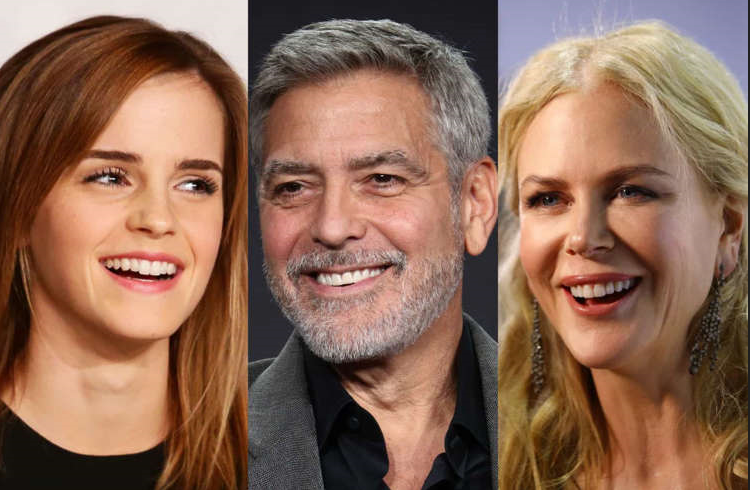This image features three closely cropped panels of well-known celebrities, each smiling broadly and showing their teeth. In the left panel is Emma Watson, with straight auburn hair and dark eyes, wearing a black shirt. She is gazing towards the right. The middle panel showcases George Clooney against a dark gray or black background, smiling warmly. With salt-and-pepper hair and beard, he dons a gray jacket over a black shirt. Finally, the right panel presents Nicole Kidman, adorned with blonde hair cascading down to her shoulders and long, sparkly earrings. She, too, is smiling and looking towards the left. All three celebrities are positioned almost directly forward, creating a harmonious triad of joyful expressions.